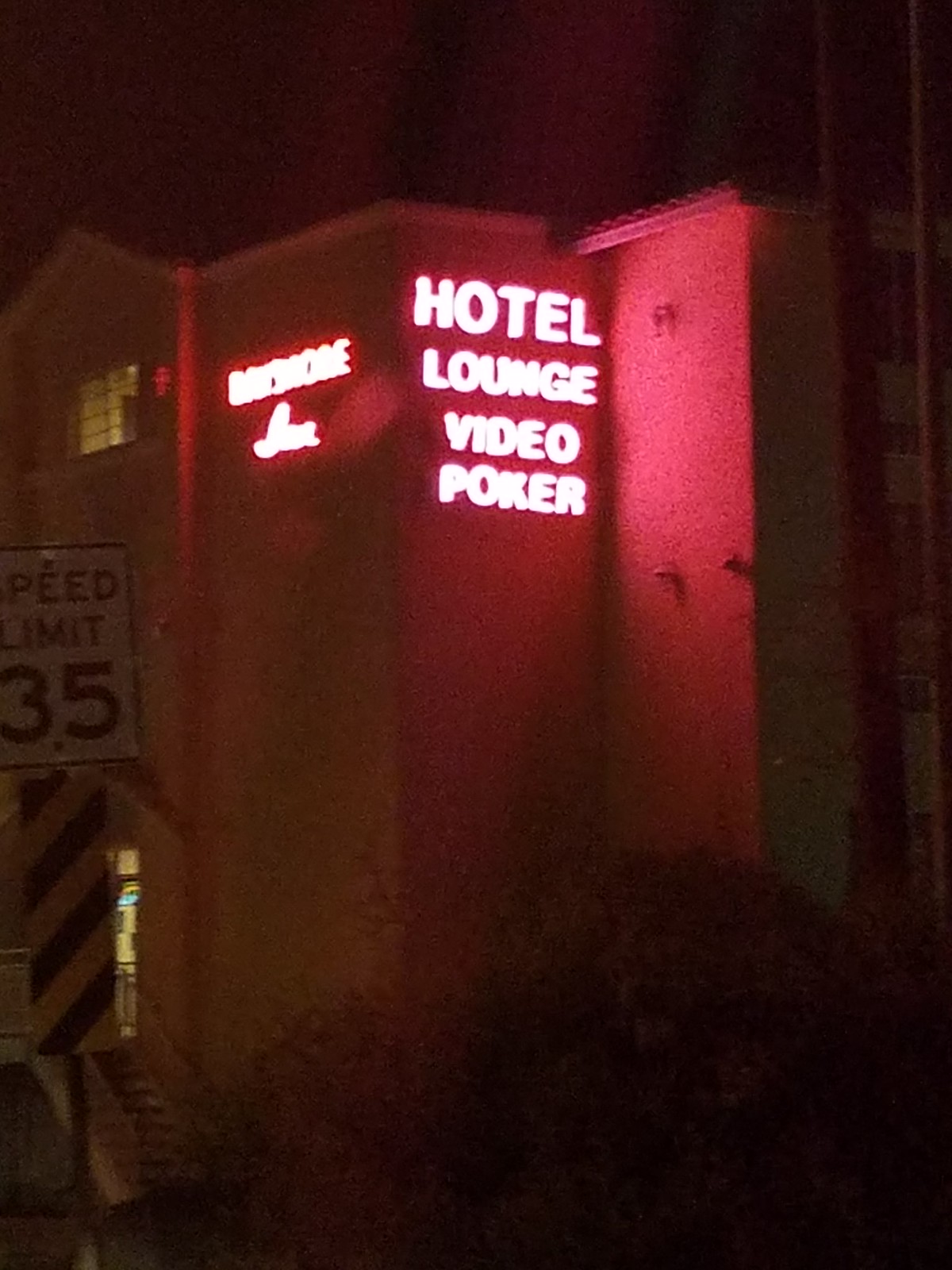The image captures the night-time exterior of a building, under a pitch-black sky that suggests it was taken during the late hours. The photograph predominantly showcases a corner of the building's facade. Dominating the scene is a vivid red neon sign, arranged in a vertical stack with the words "Hotel," "Lounge," "Video," and "Poker" sequentially positioned from top to bottom.

To the left of this neon display, there's a hint of another neon sign, though its text is difficult to decipher due to the image's slight blurriness caused by light exposure. Adjacent to the building, on the left-hand side of the image, a speed limit sign is visible, indicating a limit of 35 miles per hour. Beneath this sign, a black and yellow caution rectangle is present, adding an extra layer of visibility and alertness for passersby.